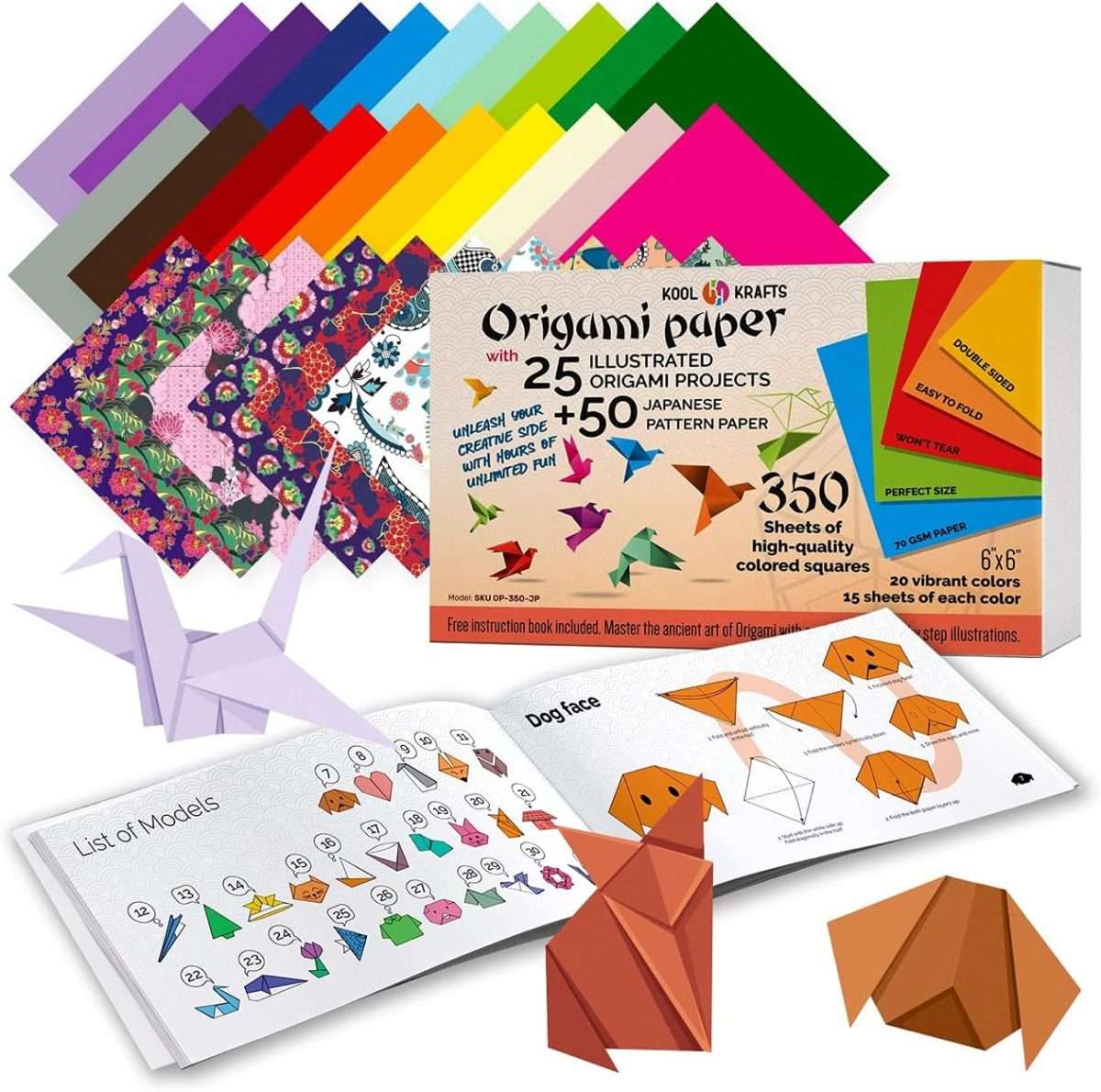The photograph is an advertisement for the Cool Crafts Origami Paper set. The set includes 350 high-quality, double-sided, 6x6 inch paper squares available in 20 vibrant colors, with 15 sheets of each color, and 50 Japanese patterned papers. It also contains a detailed instruction book featuring 25 illustrated origami projects. In the foreground, the open instruction book showcases a comprehensive list of origami models on the left page and a step-by-step dog face tutorial on the right. In front of the book, several completed origami structures, including a cat and the dog face from the tutorial, are displayed. The box, centrally positioned, highlights the product's features, promoting the ease of folding and the paper's tear-resistant quality. Behind the box, rows of colorful paper are shown: purples, blues, and greens on the top row, reds, yellows, and pinks on the second row, and floral patterned paper on the bottom row. The ad encourages unleashing one's creative side with hours of unlimited fun and mastering the ancient art of origami.